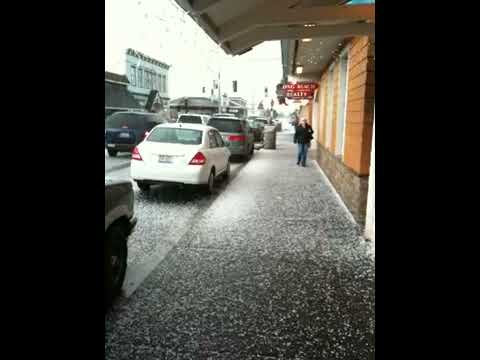The photograph captures a bustling street scene during daytime, depicting a rain-soaked sidewalk lined with orangey-brick buildings to the right. An awning overhead is dripping water, indicating ongoing rain. A solitary woman, clad in a black jacket and blue jeans, walks towards the camera amidst the wet surroundings. To the left, parked cars occupy the sidewalk's edge, and further left, vehicles are seen moving slowly, hinting at a possible traffic jam. Snow or hail covers the ground, adding a layer of white to the dark gray sidewalk and road. A red, distant shop sign stands out above the scene, though its text remains unreadable. Across the street, more buildings are visible, contributing to the urban backdrop.